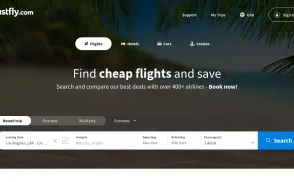The screenshot depicts a partially loaded travel website characterized by a dark blue banner at the top of the page. At the center of the page is a prominent search bar, adorned with palm tree imagery on the right side, which stands against a backdrop featuring a warm, sunny sunset glow. The website appears to focus on vacation planning and booking, offering various travel destinations. A lime green search button is positioned within the search bar, adding a splash of color. The lower section of the page showcases a series of images as recommendations or featured locations. The leftmost two images highlight water-centric destinations, while the image to the far right features an urban scene with a prominent stone building, suggesting a city destination.